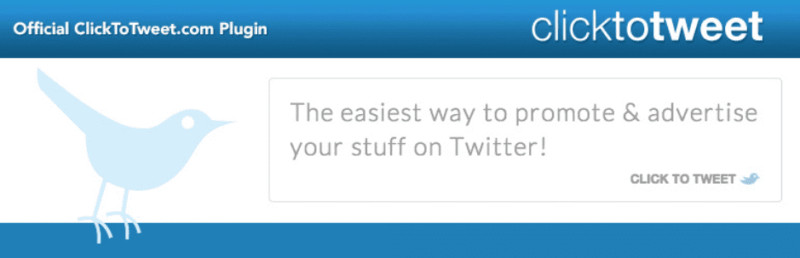This is a detailed description of a cropped screenshot showcasing a large rectangular banner for the official Click-to-Tweet.com plugin. The banner features a thick blue box running across the top and a thin blue box along the bottom, with a central background in white. A blue silhouette of a bird is positioned towards the left, standing on the lower blue box. To the right of this bird silhouette, in the center of the white background, there is a thin, gray outlined box containing the text: "The easiest way to promote and advertise your stuff on Twitter" in large gray font. In the bottom left corner of the wide, rectangular banner, bold black letters spell out "Click to Tweet," accompanied by another blue bird outline. The top left section of the banner reads "Official Click-to-Tweet.com Plugin" in bold white letters. The overall banner design is tall and very wide, emphasizing a clean, segmented layout.